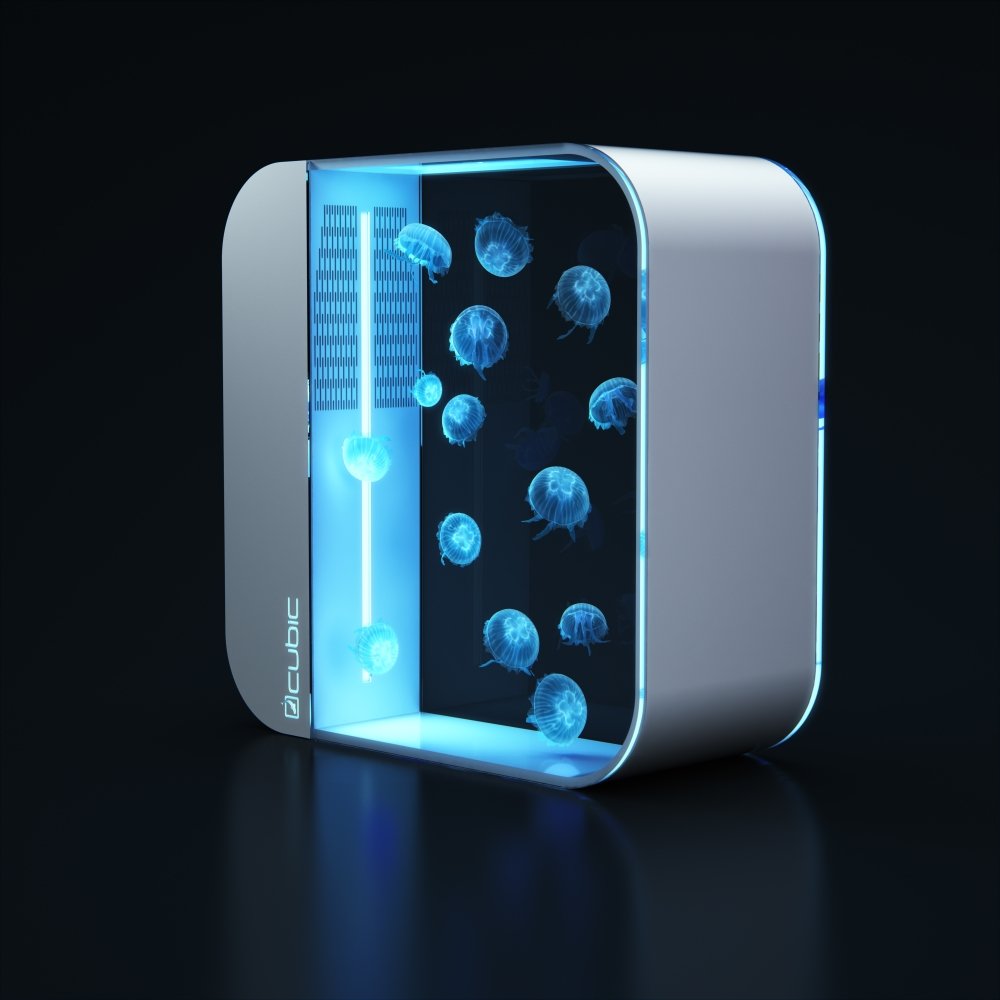The image depicts a sleek, futuristic object against a completely black background. The object has a cubic, rounded-square shape with curved, silver metallic edges. The left-hand side features a strip bearing the logo "Cubic," a technology company. Inside the object, approximately ten translucent jellyfish appear to be floating, illuminated by a soft bluish backlight that gives them a mesmerizing, almost ethereal glow. The absence of any vegetation or bubbles suggests that these jellyfish might not be real but rather a digital or holographic display. On the left side of the object, there is a small grate or vent with a blue light, possibly part of the equipment housed within the device. The overall minimalistic design, combined with the precise lighting and detailing, creates a sense of an advanced technology display, blending both art and innovation.